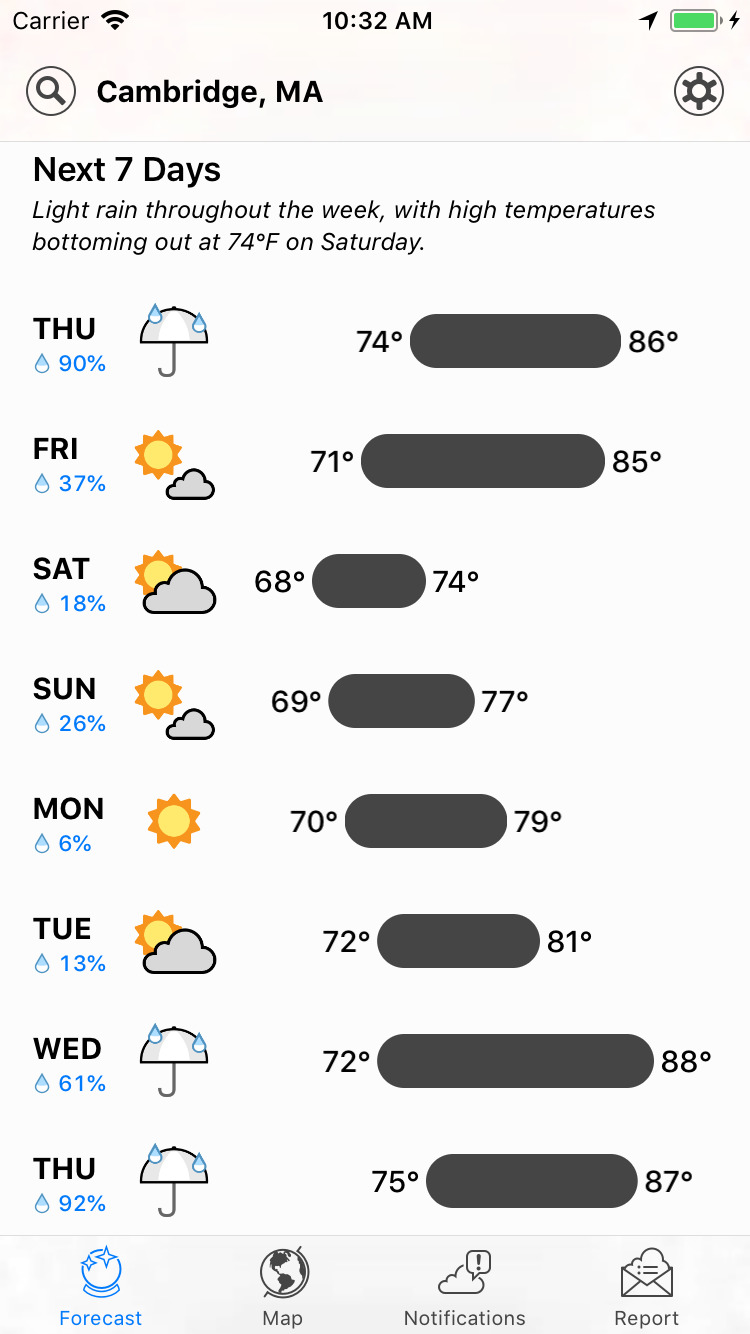The image is a screenshot from a weather app on an iOS Apple device, captured at 10:32 AM. The device shows a full battery that is being charged and is connected to the internet. The main focus of the screenshot is the seven-day weather forecast for Cambridge, Massachusetts. 

The forecast indicates consistent light rain throughout the week, with high temperatures ranging between the 70s and 80s Fahrenheit. The temperature hits a low of 74°F on Saturday. Over the weekend, both Saturday and Sunday display lows in the high 60s and highs in the mid-70s. There is a strong chance of rain on both Thursdays and the upcoming Wednesday, with a moderate chance on Friday. Friday, Saturday, Sunday, and Tuesday are expected to be cloudy, while Monday promises clear skies with no clouds, suggesting a bright and sunny day.

At the bottom of the screenshot, the app interface includes several options: "Forecast," which is currently selected; "Map"; "Notifications"; and "Report." This image portrays a simple yet comprehensive weather application designed to inform users about the upcoming week's weather conditions.